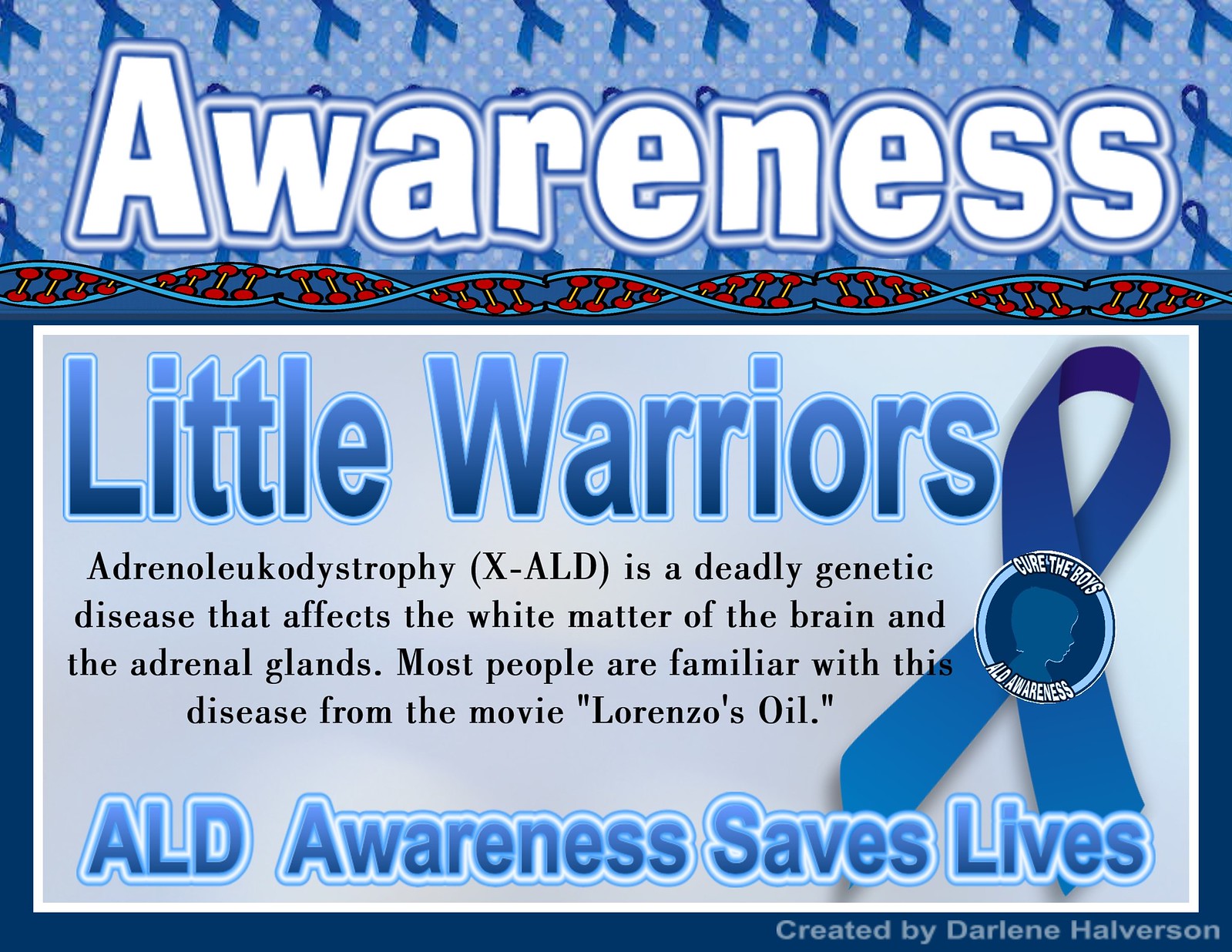This image is a digitally created advertisement with a blue-themed color scheme, featuring multiple blue ribbons in the background and playful elements. At the top, bold white text with a blue border reads "Awareness." Below this, stylized strands of blue and red DNA form part of the design. The text "Little Warriors" appears next, followed by an explanation in a Times New Roman typeface that reads, "Adrenoleukodystrophy (X-ALD) is a deadly genetic disease that affects the white matter of the brain and the adrenal glands. Most people are familiar with this disease from the movie Lorenzo's Oil." Additionally, a ribbon on the right side of the image carries the message, "Cure the Boys ALD Awareness," accompanied by a pin featuring a silhouette profile of a small boy. At the bottom, the text "ALD Awareness Saves Lives" emphasizes the ad's message. The bottom right corner includes a watermark that reads, "Created by Darlene Halverson."